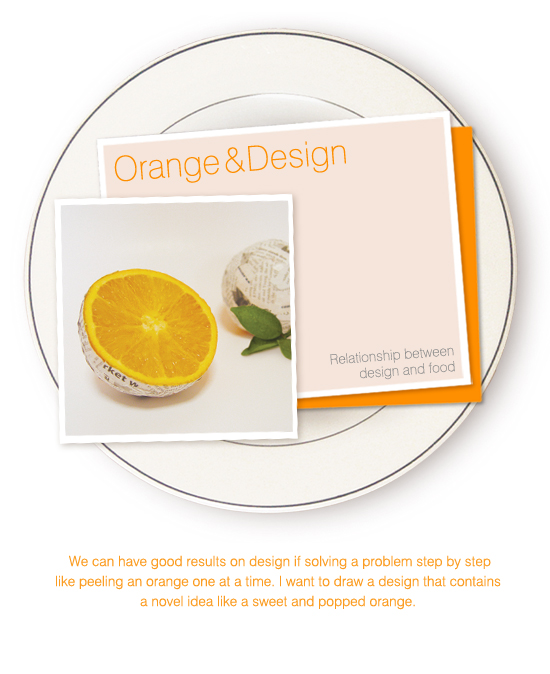The image shows a white plate as the background, featuring three layered pieces of card. The base card is orange, followed by a white card with a peach-colored background text that reads "orange and design" at the top and "relationship between design and food" at the bottom right corner. The third card on top centers an image of a halved orange wrapped in newspaper-like material, placed slightly to the left and overlapping. Additional orange text along the bottom reads, "We can have good results in design if solving a problem step-by-step like peeling an orange one at a time. I want to draw a design that contains a novel idea like a sweet and popped orange." The composition effectively plays with the theme of design intertwined with culinary elements.